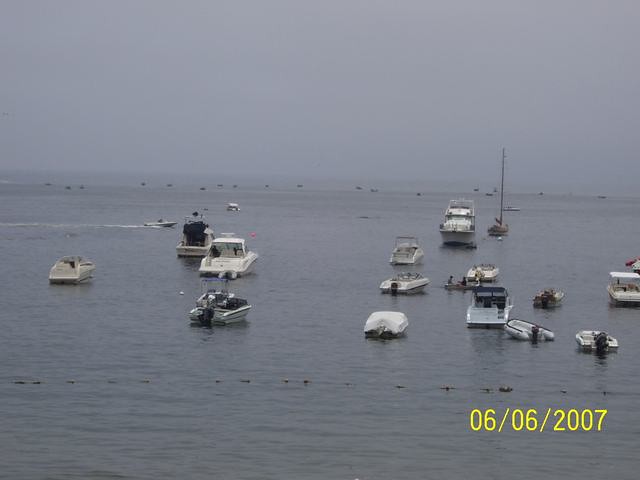This color photograph captures an outdoor scene set on a large, calm body of water under a grayish-blue sky, indicative of a cloudy day. The water reflects minimal rippling, suggesting a serene atmosphere. Scattered across the water are various types of boats, including small motor boats, speed boats, rowboats, and some with sails. A notable detail is a cluster of smaller boats located in the bottom right corner, accompanied by a life raft. The boats are all oriented with their fronts pointing towards the back of the image, and some have people aboard. In the very foreground, a few birds can be seen resting on the water's surface. Additionally, there is a date displayed in fluorescent yellow at the bottom left corner, reading 06-06-2007.